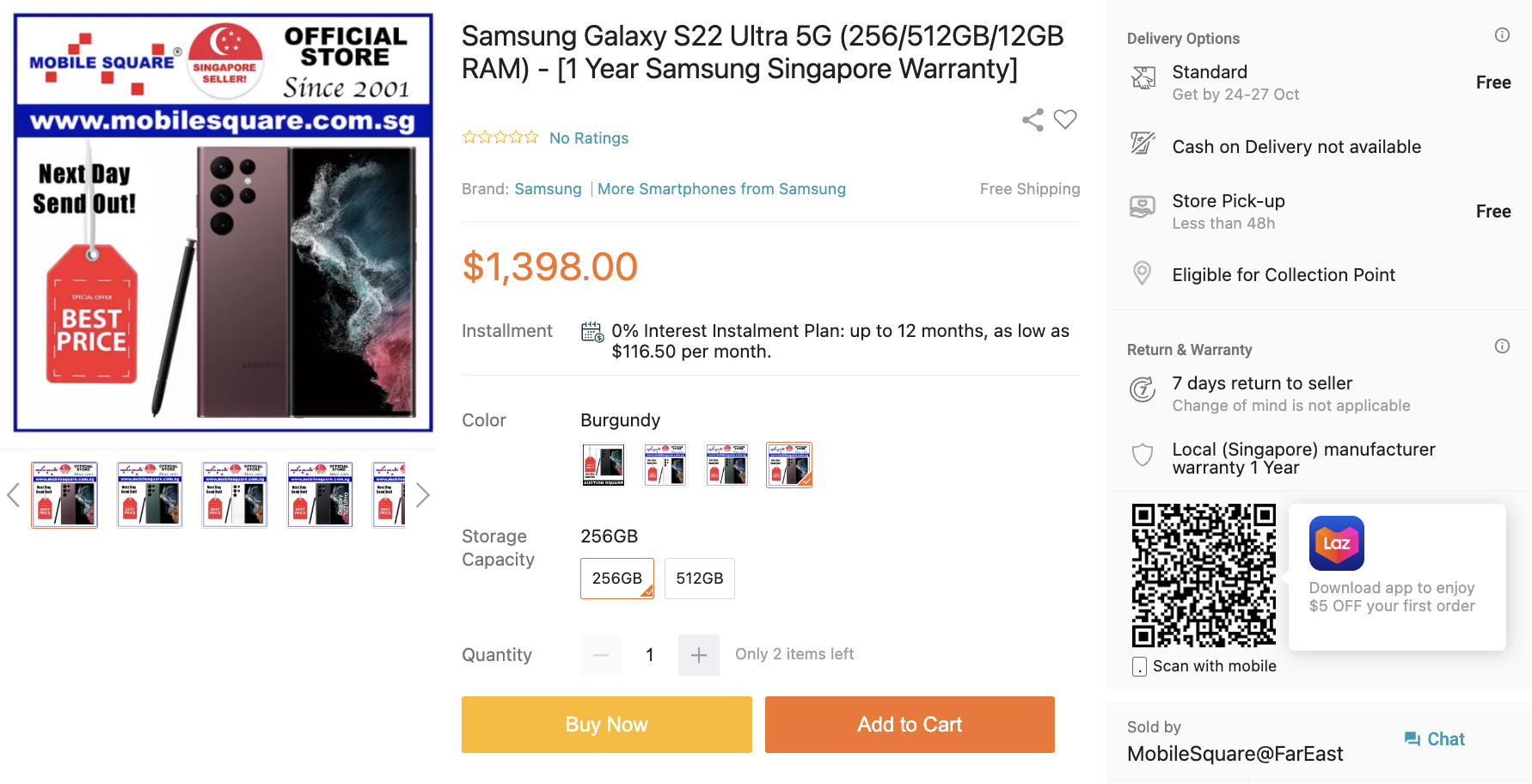The image showcases an advertisement from the official Mobile Square Singapore store, established in 2001, as detailed on their website mobile-square.com.sg. The ad features their promise of next-day dispatch and competitive pricing. 

The focal product is the Samsung Galaxy S22 Ultra 5G, available in two storage capacities: 256GB and 512GB. The highlighted model in the ad has 256GB of storage, accompanied by 12GB of RAM. The phone is covered by a one-year Samsung warranty specific to purchases in Singapore.

Displayed prominently are the following details:
1. Price: $1,398
2. Installment options: Zero interest plan for up to 12 months, starting at $116.50 per month
3. Color: Burgundy

The advertisement includes navigation options to view additional related advertisements, indicating that viewers can explore up to four and a half other offers. 

Customers have the option to "Buy Now" or "Add to Cart," with a noted delivery timeframe for the standard free delivery, expected between October 24 and October 27.